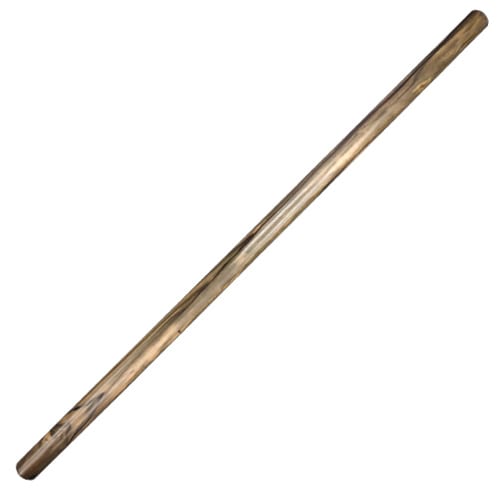The image depicts a simple, smooth cylindrical stick or rod that extends diagonally from the lower left to the upper right. This stick, which closely resembles a large wooden dowel or a standard shower rod in terms of proportion, is about 12 to 15 inches long and roughly as thick as an adult person's finger. The stick appears to be crafted from wood or has a wood-like finish, characterized by a polished texture with visible wooden grain lines and swirly patterns in lighter shades. The coloration transitions from darker brown at both ends to a slightly lighter, shinier area in the middle due to reflected light. The stick's surface is smooth with no visible shadows in the image, making it a simple yet visually distinct object.